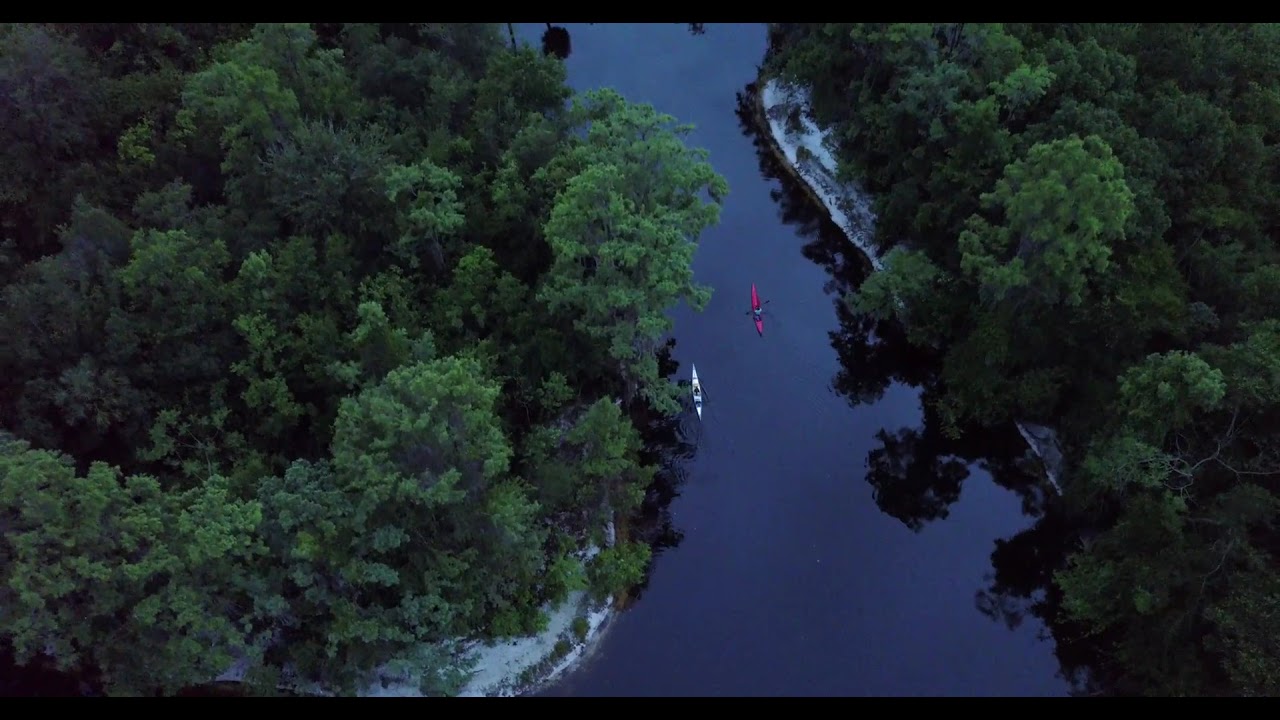This aerial photograph showcases a captivating scene of a river winding through a lush forest. The river, with its dark blue and reflective surface, slices vertically down the center of the image, flanked by dense clusters of towering green trees on both sides. In the middle of the river, two canoes – one red and one white – can be seen with people rowing. Near the water’s edge, there are sandy or possibly white structures that may be buildings or roads. The scene is captured in the late afternoon, with a darkish tone setting in, suggesting the approach of dusk. The background fades to black borders, framing this tranquil and picturesque moment in nature.